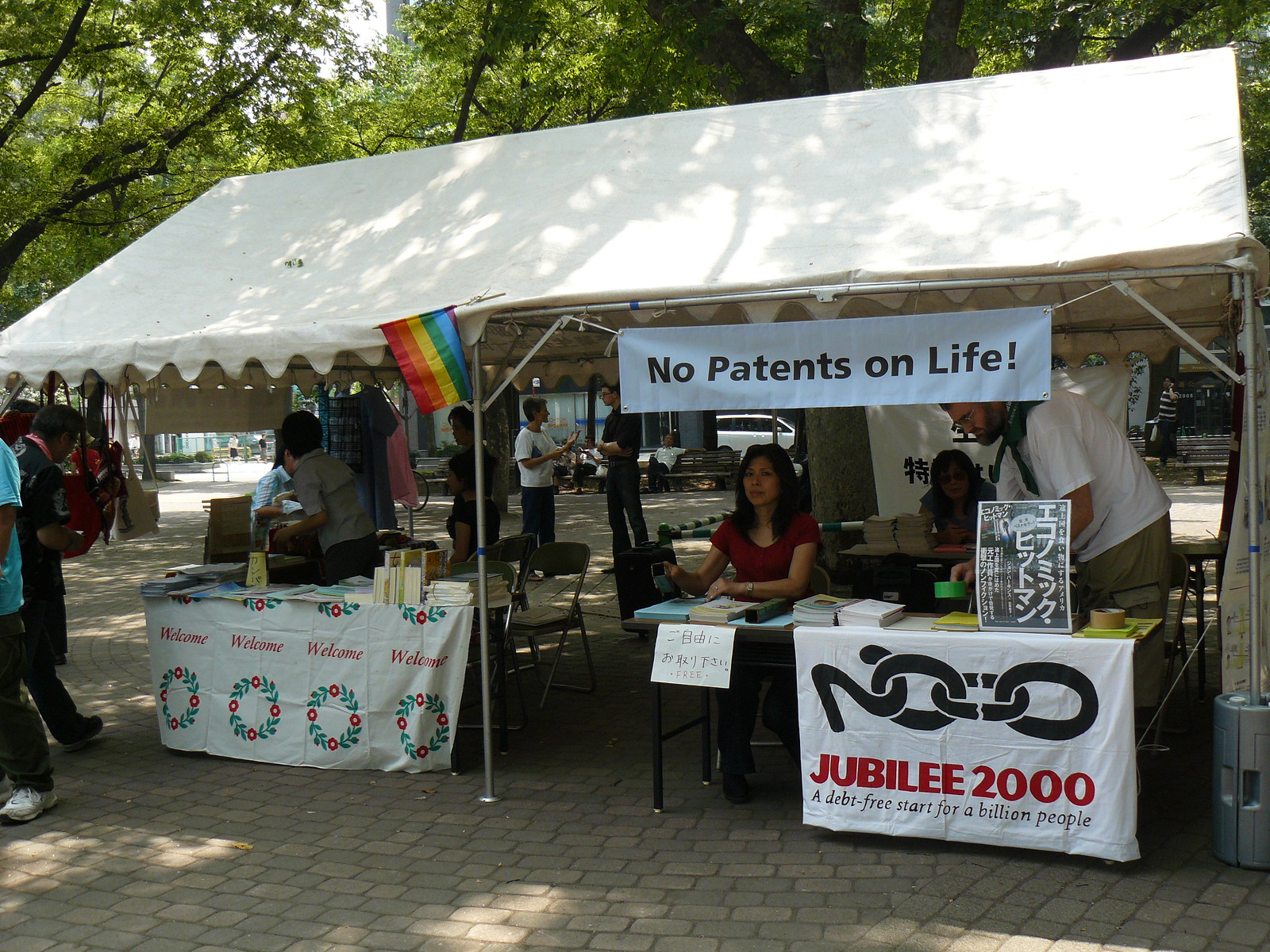The photograph captures an outdoor scene featuring several stands underneath a large white cloth tent. The tent, supported by a central pole, shelters two main booths arranged side by side. The ground appears to be paved with tiles that resemble bricks. Behind the tent, lush trees stretch in from the left and the background, harmonizing with the light sky.

On the left, there is a booth with a table covered in a cloth adorned with red writing and some wreaths beneath it, although the exact items on the table are unclear. A woman with shoulder-length dark hair in a red shirt sits here, positioned behind a small, illegible sign. To her right stands a man in a white shirt, gazing downwards.

The right booth features a prominent banner displaying black symbols with "Jubilee 2000" in red beneath it, along with smaller black writing that includes the phrase "a debt-free start for a billion people." The table itself is laden with pamphlets and booklets. This booth draws attention with its banner that reads "no patents on life" at the top. Between the two booths, a pride flag is visible.

In the broader context, the area has a college fair atmosphere, with various people milling about, some partially leaving the frame to the left. Above the entrance in the distant background, a banner spans, welcoming attendees. The whole scene exudes a feeling of community engagement, set against the lively backdrop of bustling participants and vibrant greenery.